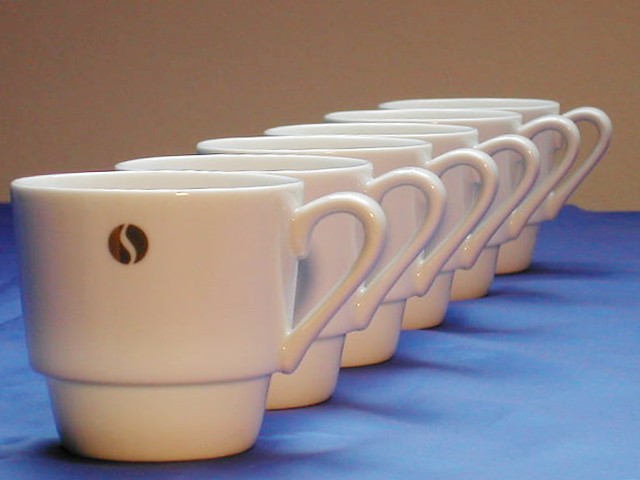This photograph showcases a precise arrangement of six white, glossy coffee mugs, possibly made of porcelain or ceramic, aligned in a perfect row from the front left corner to the bottom right corner of the image. Each mug's handle is uniformly pointed to the right. They are set against a navy blue or royal blue tablecloth, with a slightly off-white, almost eggshell, background wall. The mugs cast consistent shadows towards the bottom right.

The foremost mug displays a distinctive symbol that mirrors a yin-yang shape but features a unique design: two dark brown segments with black dots at their widest parts. The cups appear empty, suggesting this is a polished product display, potentially for a set being sold. The absence of text ensures the focus remains on the mugs' orderly presentation and the intricate emblem on the lead mug.